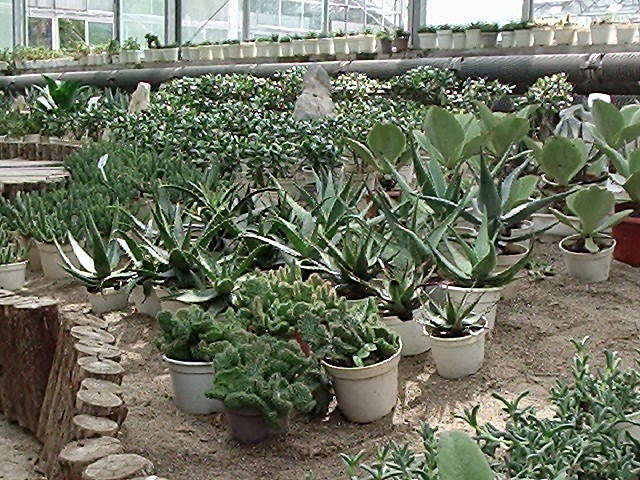The photograph showcases a vibrant nursery, likely inside a greenhouse, as evidenced by the large glass windows in the background that allow ample light to flood the space. Rows of shelves filled with small potted plants line the back, each plant housed in uniform white pots. The top shelf displays a neat array of these smaller pots, predominantly showing green leaves of various succulents and cacti.

In the foreground, larger white pots are arranged on the dirt ground, holding a diverse collection of bigger plants, including tall aloe vera, robust cacti, and broad-leaved varieties. These bigger pots seem to dominate the lower middle section of the image with their lush green foliage. 

To the left, a rustic element is introduced by a small fence constructed from vertically stood wooden logs, serving as a barrier or decorative element alongside a walkway formed with wooden planks. Below the plants in the background, a metal pipe extends horizontally, subtly framing the scene.

The overall setting is an organized and well-lit space dedicated to nurturing a myriad of green plants, predominantly succulents and cacti, all meticulously arranged in white pots on both shelves and ground, creating a tranquil and orderly environment within this vibrant nursery.